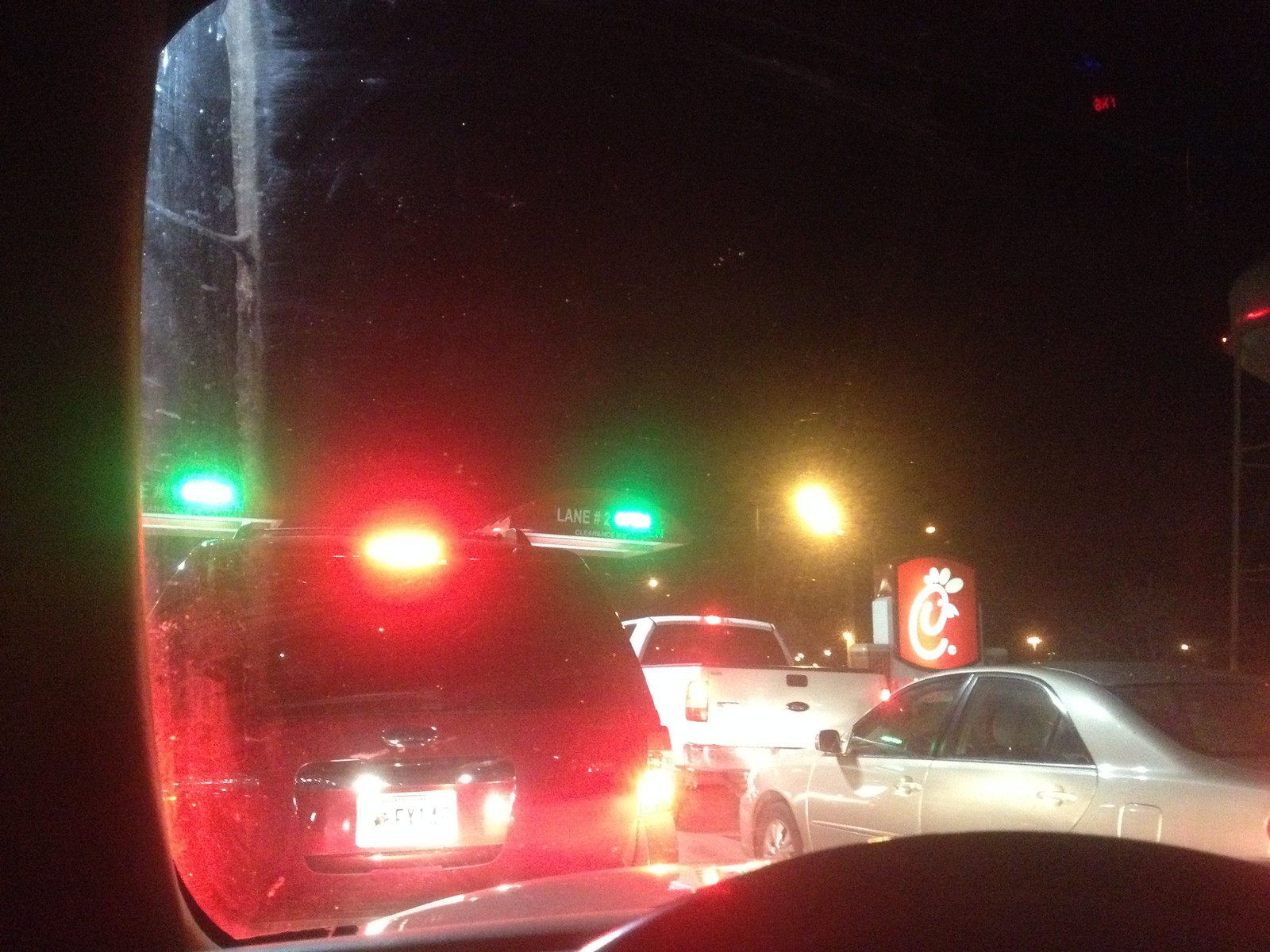The photograph captures a nighttime street scene featuring the recognizable elements of a Chick-fil-A drive-thru. Dominating the right side of the image is the red and white Chick-fil-A logo. Below the sign, a white Ford truck is parked, followed closely by a silver car that appears to be a Toyota. The scene is framed by a window, possibly from the perspective inside a vehicle, marked by a light bar with two green lights flanking a single red light in the center. Near these indicator lights, a red vehicle is partially visible, though its license plate is blurred, and further details are obscured by the dim lighting. The overall darkness suggests that the photograph was taken late in the evening or at night. The slight reflection of the dash cam in the window indicates that the image was captured from inside a vehicle within the Chick-fil-A drive-thru, capturing a snapshot of the late-night ambience.